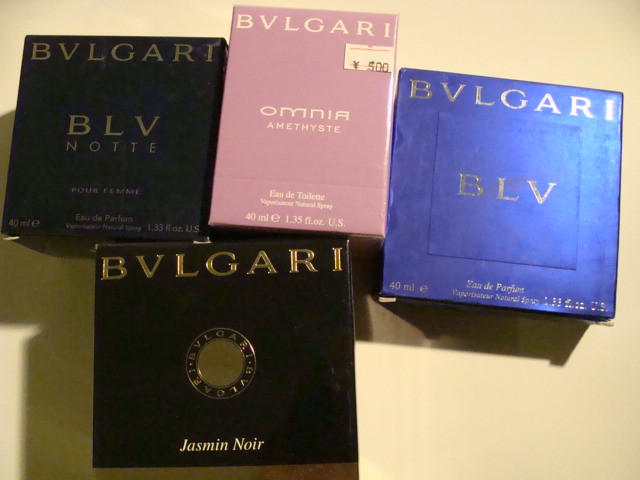The image depicts four elegant boxes from the luxury brand BVLGARI, arrayed on an off-white yellow surface. Each box, showcasing different BVLGARI fragrances, is distinct in color and inscription. The upper left box is sleek and black, adorned with gold text reading "BVLGARI BLV Notte," and further specifies "Porfem" along with a possible indication of "40 milliliters." To its right, the second box is a delicate pink, featuring white text that spells out "BVLGARI Omnia Amethyst," denoting "Eau de Toilette," and a price tag of 500 yen. This box also mentions "40 milliliters" or "1.35 fluid ounces US." The next box to the right is a striking blue, marked with "BVLGARI BLV" and "Eau de Parfum," and similarly notes "40 milliliters." Lastly, the lower black box has a central circular design with the name "Jasmine Noir" written at the bottom. While the blue box has a shiny surface that reflects light, the other boxes exhibit a more matte finish.